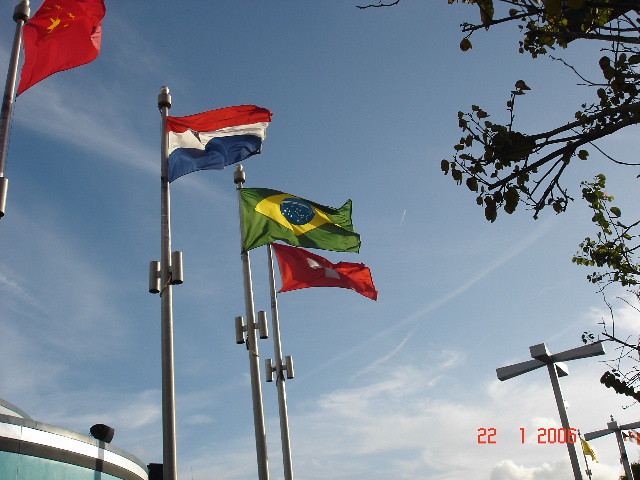In this vibrant outdoor photograph taken on January 22, 2006, we are looking up at a series of flags from different countries, mounted on intricately designed metal flagpoles resembling an "H". From left to right, the first flag in the upper left corner is predominantly red with a touch of yellow, likely bearing yellow stars. Next to it, about a quarter of the way to the right, is a flag with horizontal stripes of red, white, and blue, resembling the French flag. The third flagpole proudly supports the Brazilian flag, identifiable by its green background, yellow diamond, and blue circle with white details. The fourth flag, slightly set back, is also red with white splashes at its center. The blue sky provides a serene backdrop, adorned with wisps of white clouds and a few tree branches peeking in from the upper right. The lower right corner of the image displays red text overlay reading "22 1 2006" and also features some narrow streetlamps, as well as a hint of a semicircular roof of a building in the lower left corner.